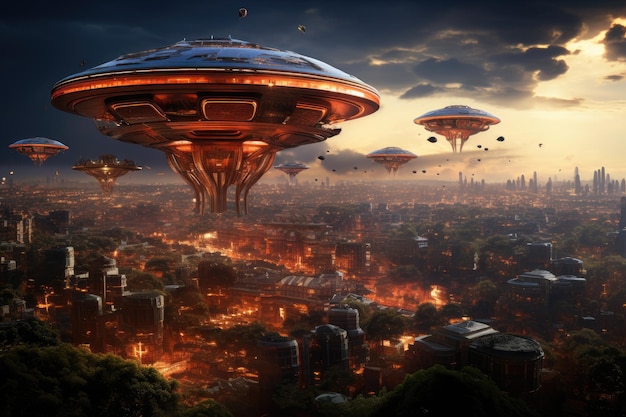The image depicts a scene, possibly computer-generated or a 3D rendering, of an alien invasion taking place over a city at dusk or dawn. The cityscape features medium-height buildings in the foreground and distant skyscrapers creating a layered skyline. The sky, dominated by thick, dark grey clouds, occupies three-quarters of the image. Bright, orangey-red flames engulf the lower sections of the buildings, illuminating the scene dramatically.

Hovering ominously above the city are several mechanical, mushroom-shaped flying saucers. The closest spacecraft appears in intricate detail, showcasing a blue mechanical top that slopes downward, giving it a characteristic UFO appearance, while the underside glows in a rust-colored hue. These alien vessels feature dangling appendages reminiscent of squid tendrils. There are at least five to six of these saucers vividly portrayed, with more shadowy figures in the background, emphasizing the vast scale of the invasion. The combination of the fiery cityscape, the menacing UFOs, and the stormy sky creates a scene reminiscent of a high-stakes, cinematic moment out of a Marvel movie.